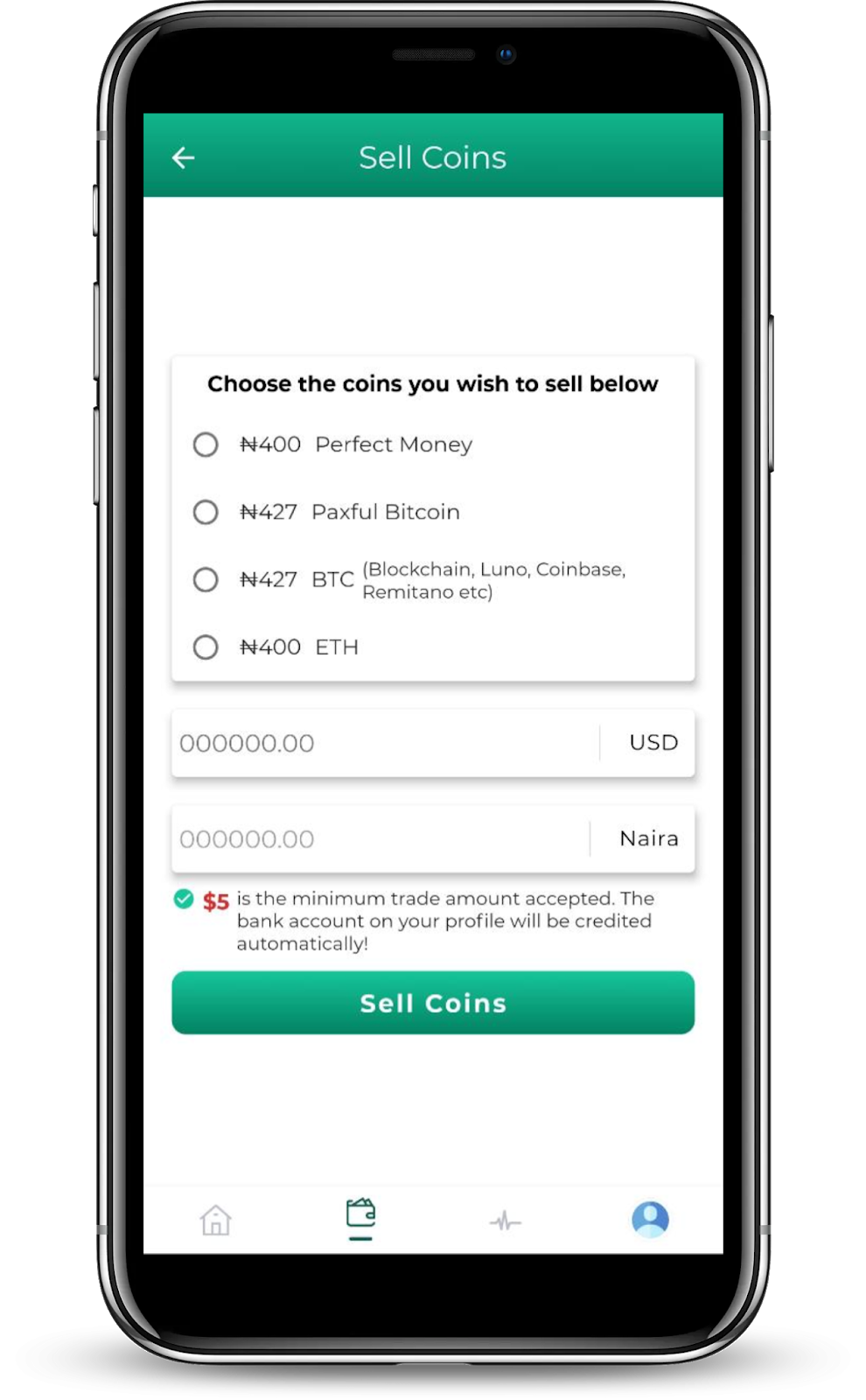The image showcases a mobile interface for a cryptocurrency trading application or website. 

At the very top, there's a green border, and situated on the far left within this border is a white arrow. Centered within the green border, the header reads "Sell Coins" in clear, bold text. 

Just below the green border, a prominent white field displays a rectangular box with the text, "Choose the coins you wish to sell below," written in black. Within this space are four options listed in gray:
1. "400 Perfect Money"
2. "427 Paxful Bitcoin"
3. "427 BTC or Bitcoin"
4. "400 Ethereum ETH"

Further down, there's a section labeled to input "Amount you want to sell in USD" followed by a text box pre-filled with "NARA". 

A small note beneath this text box informs users that the minimum trade amount accepted is five dollars.

Finally, positioned at the bottom of the interface is a green button with the label "Sell Coins," which users can select to initiate their transaction.